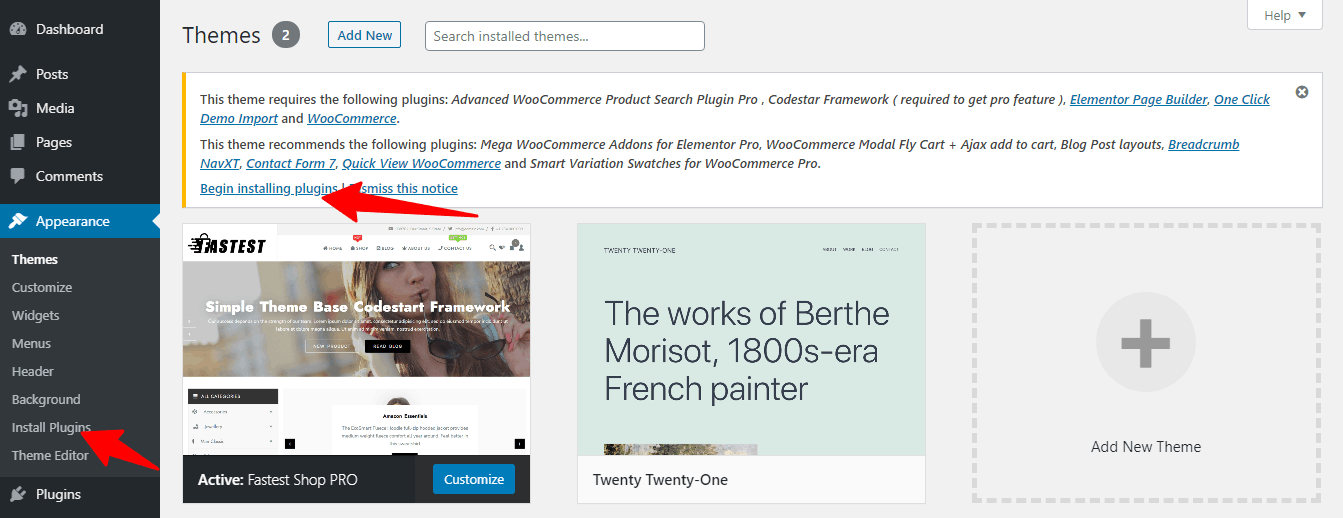The image displays a website's dashboard interface, typically seen in content management systems like WordPress. 

On the right side, there is a black and white sidebar featuring menu options: "Dashboard," "Posts," "Media," "Pages," "Comments," "Appearance" (highlighted in blue), "Themes," "Customize" (with sub-options: "Menus," "Header," "Background"), "Plugins" (marked with a red arrow), "Theme Editor," and "Plugins" again. The background transitions to gray.

At the top of the sidebar, "Themes" is written in black alongside a gray circle containing the number "2." Below this, in blue text, reads "Add Note" followed by a white search box with light gray text that reads "Search themes...".

To the left, a content section is visible, bordered by a vertical orange strip on the left side. The message in black text states, "This theme requires the following plugins: Advanced Rule, WooCommerce Product Search Plugin Pro, CodeStar Framework (required to get Pro features)." Additional required plugins are listed in blue underlined text: "Elementor Page Builder," "One Click Demo Import," and "WooCommerce."

The message continues in black text, "This theme recommends the following plugins: Maker WooCommerce Add-ons for Elementor Pro, WooCommerce Modal Fly Cart, Ajax Add to Cart, KBlog Post Layouts," followed by "Breadcrumb Beacon" in blue underlined text. A red arrow points to this section, obscuring some words.

At the bottom, black text references "The work of Berthe Morisot, 1800s-era French painter," followed by a date range: "2020-1."